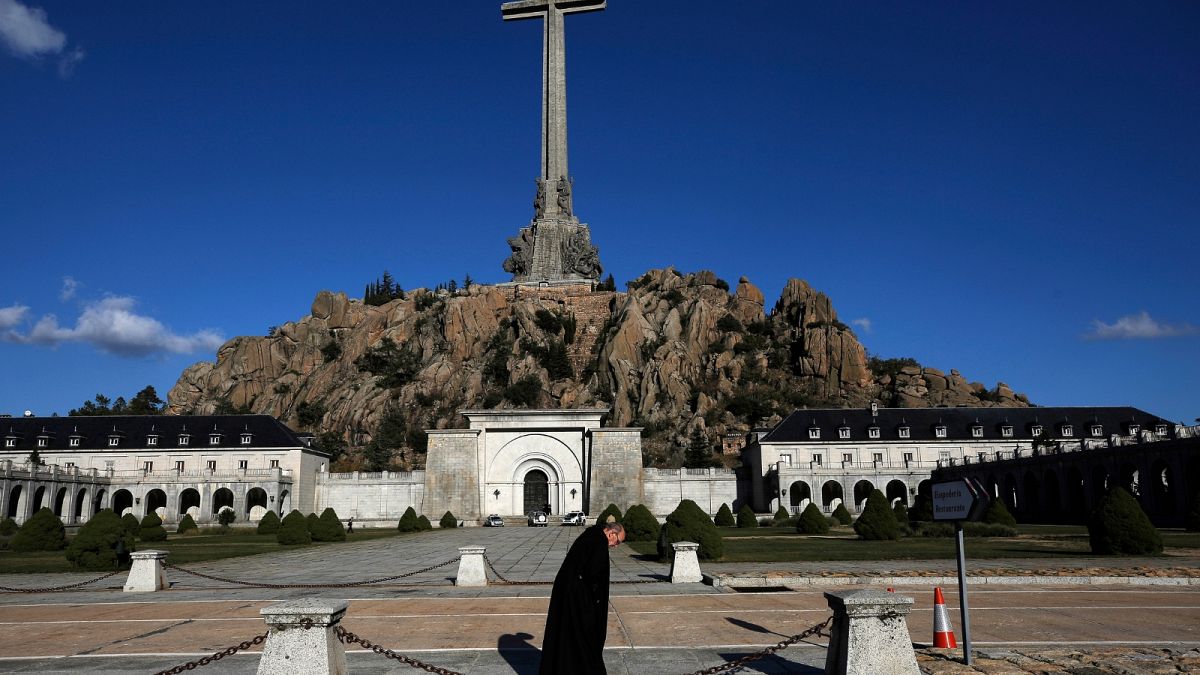In this detailed outdoor, daytime photographic image, a large gray concrete cross dominates the scene, perched majestically atop a cliff intertwined with trees and rocks. Below the cliff, there is an elaborate religious monument comprised of three distinct sections featuring arched entrances, gray gabled roofs, and intricate architectural details that suggest a monastery or church. The buildings are made of granite and exhibit a meticulous design, fortified with small concrete pillars capped with pyramid tops, connected by brown chains.

In the foreground, a priest or monk, an elderly white man donning a black robe and glasses, walks with his head down, moving from left to right across a red-brown paved walkway. This walkway is bordered by a gray stone path that leads to the monumental buildings. An orange and white traffic cone and a blurred sign, with some illegible text possibly containing an "R" and an "E," add modern-day elements to this historically rich setting.

The background showcases a rocky hillside leading up to the enormous cross, against a strikingly rich blue sky scattered with a few gray or white clouds, adding a serene yet powerful contrast to the monumental religious site. The entire scene evokes a sense of tranquility and reverence, symbolizing the intersection of nature, spirituality, and human craftsmanship.